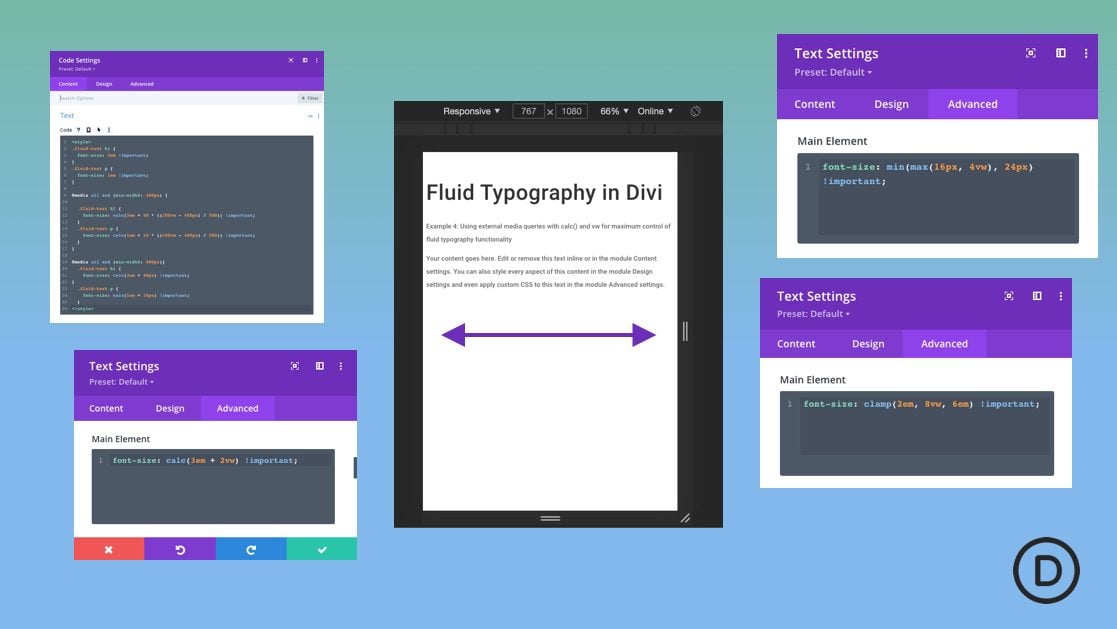The background of the image features an ombre gradient that transitions from green at the top to blue at the bottom. Four boxes are aligned around a central purple box, with two boxes on each side. 

**Left Side Boxes:**
- The first box at the top left has a purple header and contains partially legible text including "code settings."
- The second box underneath it also has a purple header and mentions "text settings" with "preset default" visible upon zooming in.
- Three tabs are visible titled "Code," "Design," and "Advanced." Beneath these tabs, the text "main element" is displayed in black.

**Right Side Boxes:**
- The top right box has a purple header with the text "text settings" and "preset default." It includes sections labeled "Content," "Design," and "Advanced," followed by the phrase "main element" in black.
- The second box underneath mirrors the same text and layout as the one above it, both featuring "text settings," "preset default," "Content," "Design," "Advanced," and "main element."

**Center Box:**
- A central black rectangle features white text at the top, displaying "Responsive: 761 by 1080, 66% online."
- Inside this rectangle, a white section with black text reads "Fluid Typography" followed by "DIVI Typo."

This detailed caption aims to convey the visual arrangement and text content more clearly.